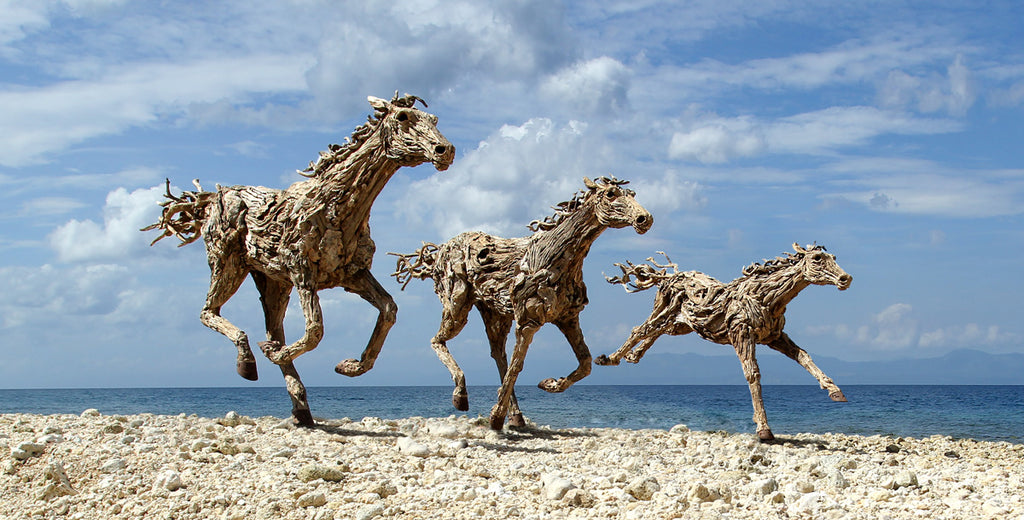The image portrays a captivating coastal landscape with a bright blue sky filled with scattered white clouds, extending down to meet a body of water on the horizon. Below the water, a rocky sandy beach stretches across the scene. Central to the composition are three intricately crafted sculptures of horses, seemingly carved from driftwood or beechwood. These wooden sculptures arranged from right to left present a dynamic scene of galloping horses in mid-motion, as though they were genuinely running across the beach. The largest horse, positioned on the right, has three legs in the air and appears the most forward, with its tail streaming behind as if caught in the wind. The middle horse, slightly smaller, also exudes movement with two legs on the ground and two lifted. The smallest horse on the left, resembling a young foal, has one front leg touching the ground and displays shorter legs, completing the visual suggestion of a family unit—likely a male, a female, and their offspring. The natural wooden texture and detailed craftsmanship capture a vivid sense of life and motion, blending seamlessly into the tranquil and picturesque seascape.